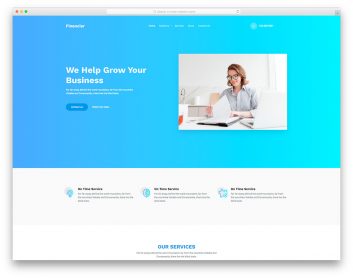The image features a woman with short brown hair and glasses, seated at a desk. She is wearing a light gray collared shirt and has a large notebook in front of her. The background is divided into two main colors: the upper section is bright blue, and the lower portion, including the wall behind her, is completely white. 

In the upper left corner, there is a search bar accompanied by three small circles in red, yellow, and green, reminiscent of typical window control buttons. To the left of the woman, in bold white text, is the phrase, "We can help grow your business." Below this, there are three clickable areas, each marked with a blue circle and accompanied by subheadings in black text. However, the content within these areas is too small to read. 

At the bottom of this section, in large blue bold text, the phrase "Our Services" is clearly visible. Below this heading, there are two rows of small, unreadable black text. The overall design suggests a professional and business-oriented theme, with important messages and navigation options highlighted in blue and white.